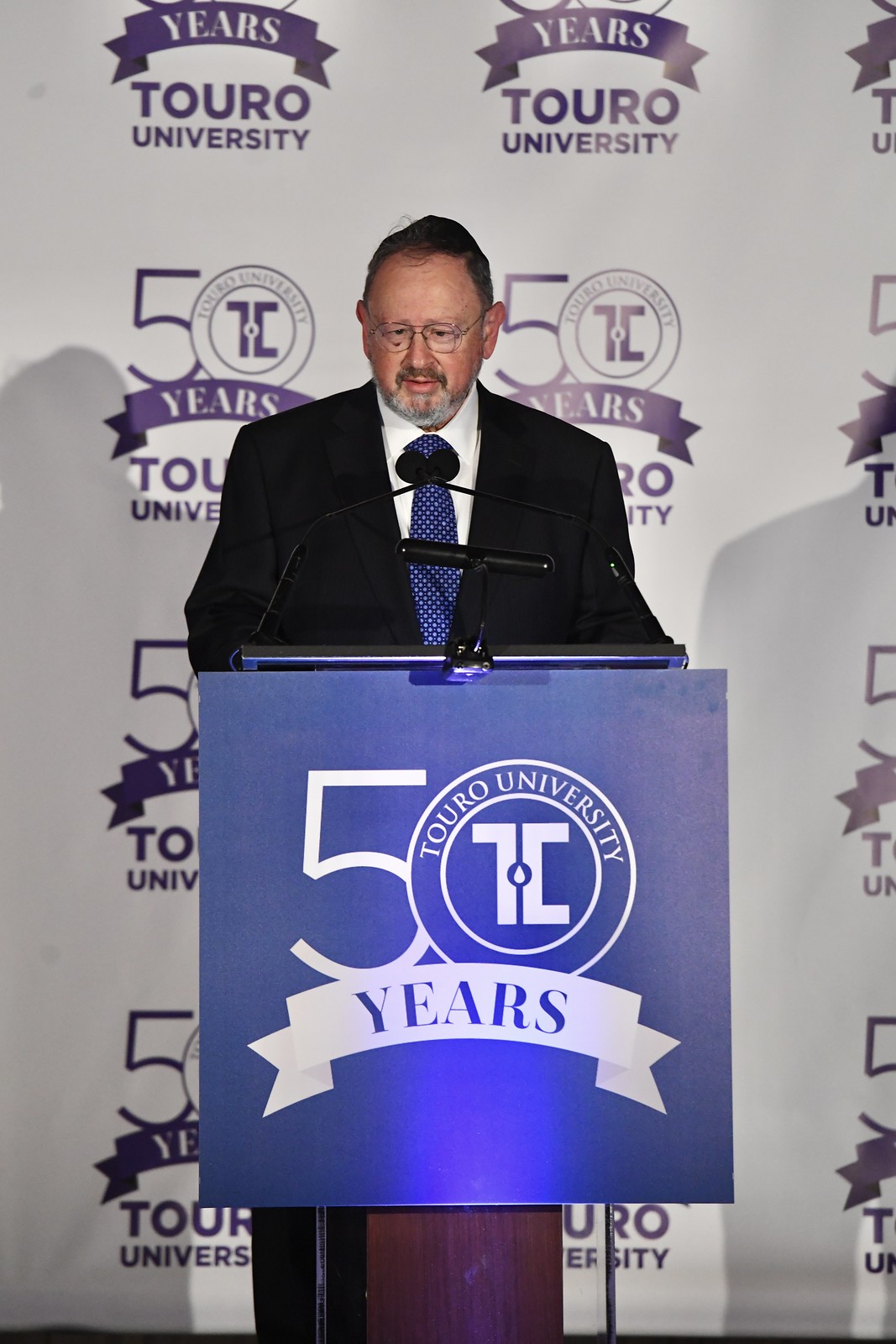In this vertically aligned rectangular picture, an older gentleman is standing at a dark brown podium, speaking into two microphones. The podium features a prominent blue sign with a large white "5" and an "O" formed by two circles, inside which it says "Touro University." The man is dressed in a black suit jacket, a white collared button-down shirt, and a blue tie adorned with tiny white dots. He has wire-rimmed glasses, a receding hairline, short brown hair, brown mustache, and partially gray facial hair. Behind him, the backdrop is a white wall with recurring purple text that reads "Touro University, 50 years."